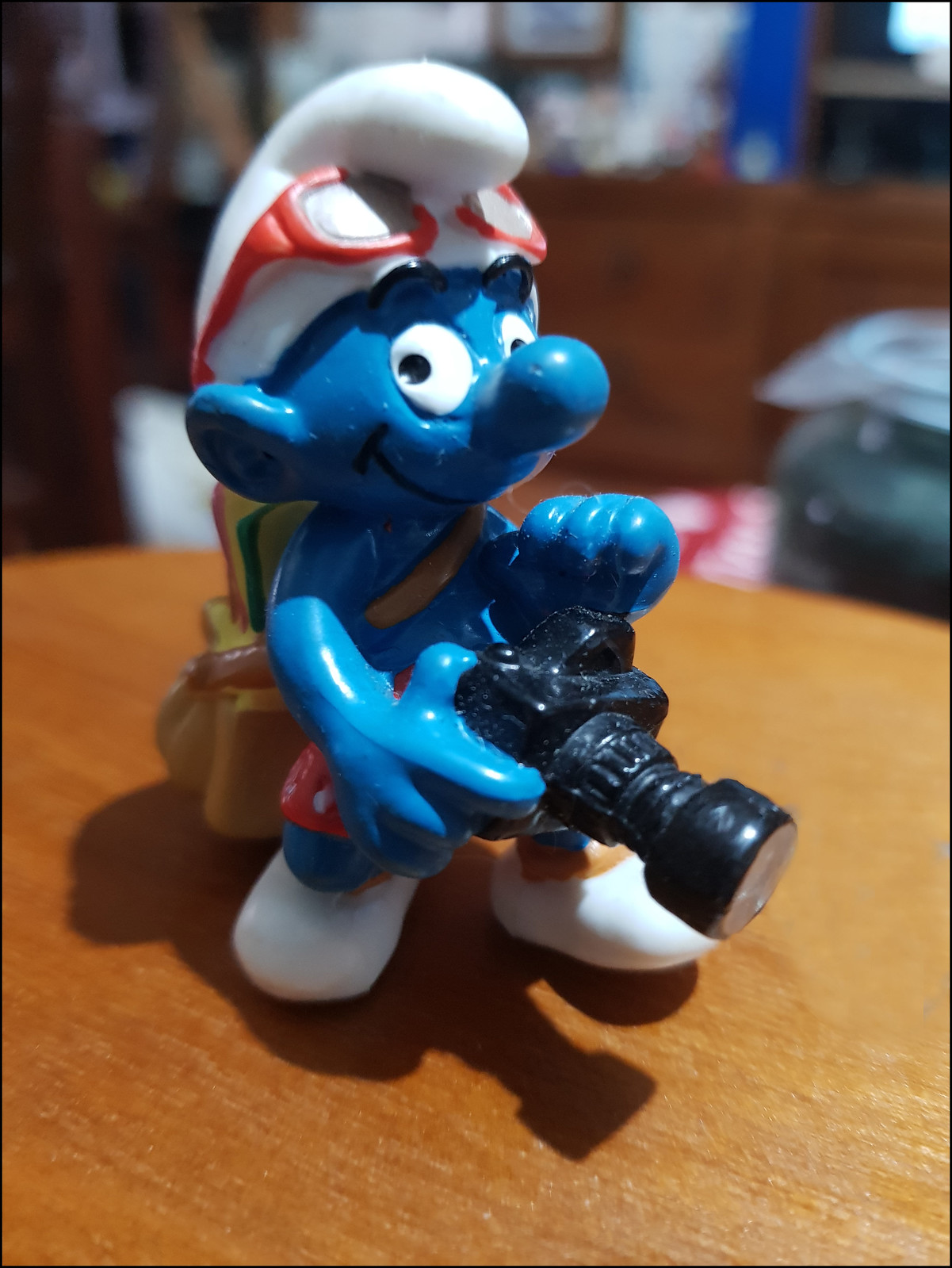In this photo, there is a small, highly detailed blue Smurf figurine placed indoors on a round wooden table. The Smurf is dressed in a white conical hat topped with red-framed glasses and white shoes. The figurine is smiling, showcasing its big round eyes, round bald nose, and large ears, giving it a very animated and cartoony appearance. The Smurf is holding a small black camera with a long lens, adding to its charming and engaging look. Additionally, the figurine is equipped with a brown, yellow, and green backpack slung over its shoulder, filled with various items. The scene is well-lit from above, casting distinct specular highlights. In the background, the room appears to have brown cabinets, papers, some debris, walls, and a window, all of which are blurred out, drawing focus to the intricately designed Smurf figurine.